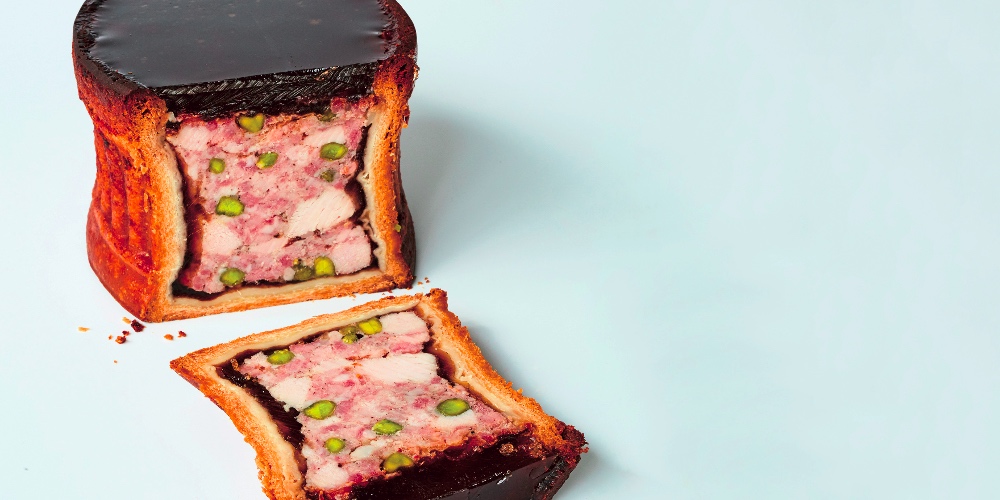This photograph showcases a partially sliced baked meat pie, placed against a baby blue background. The pie, originally a cylindrical, drum-shaped form approximately four inches in diameter, features a deep brown crust with a jet-black top. One vertical slice has been cut and laid flat on a white surface, revealing the dense, cohesive filling inside. The filling, which appears to be a pinkish meat mixture resembling corned beef hash, includes visible white fat and scattered green bits that could be pistachio nuts or peas. The meat has slightly pulled away from the crust during baking, creating a small gap between the filling and the crust. Crumbs from the cut are evident around the base of the pie and on the surface.